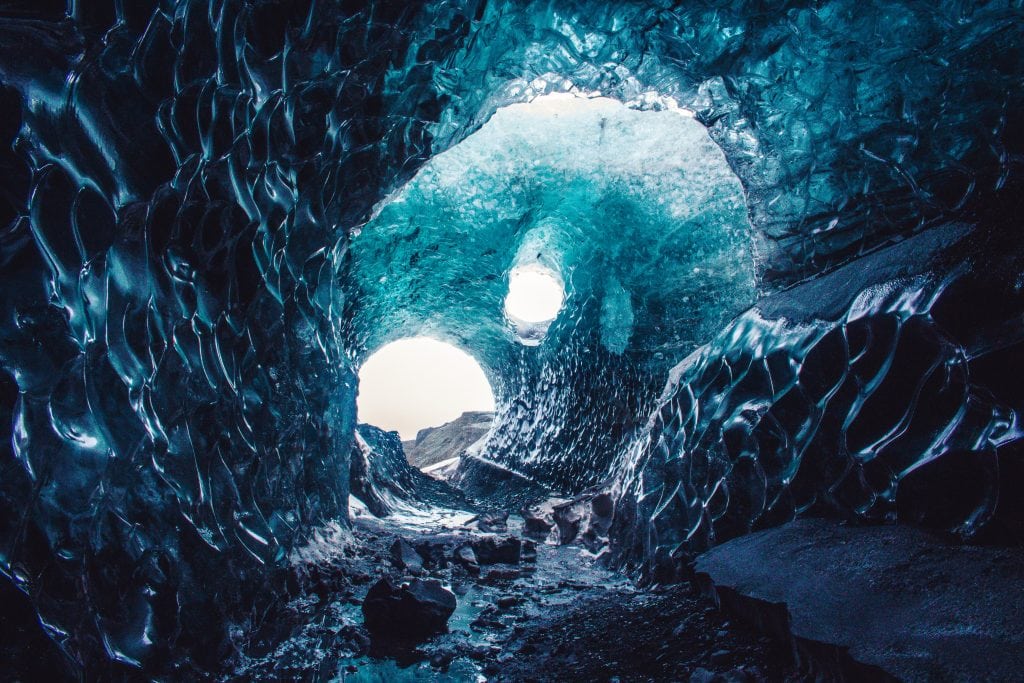The image portrays an icy cave that resembles a massive, oceanic wave frozen in time. The cave walls, rippling with texture, mimic a substantial wave that might project overhead, gradually crystallized in mid-air. The color palette shifts from dark ocean blue in the foreground to lighter tones toward the cave's exit. This exit comprises two apertures: a higher, window-like hole, and a lower entrance that forms a nearly perfect circle, allowing light to filter through and brighten the scene. The ice retains its wave-like formation throughout, even in the areas more exposed to light, enhancing the sense of an augmented reality or fantasy-like environment. The cave floor appears shallow and scattered with some rocky material, emphasizing the illusion of a wave caught in motion.